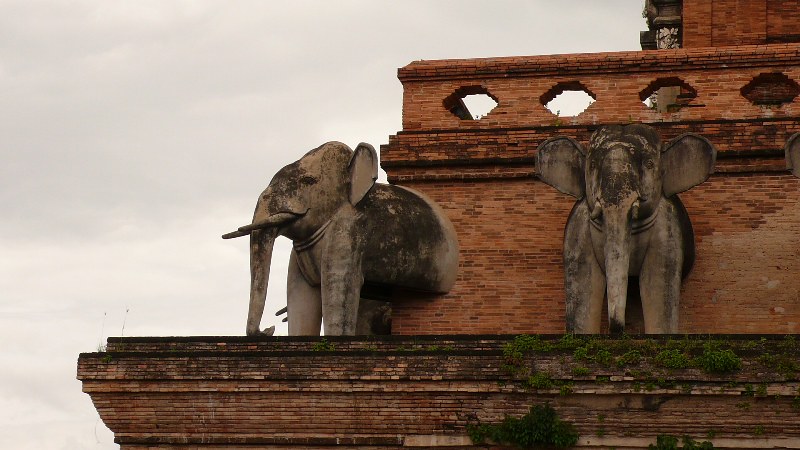The photograph captures the upper corner of an old, reddish-brown brick building with distinctive architectural details, suggesting it might be from another country. The sky is overcast, adding a hazy, somewhat somber mood to the scene. Prominently featured are three large, gray, weather-worn elephant statues emerging from the brickwork. The two most visible elephants, positioned near the corner of the building, display their trunks, tusks, ears, and front legs, seemingly poised in motion. The brickwork above and around the elephants includes decorative elements such as football-shaped openings and a plateau-like structure. The entire building facade appears aged, with dirt, dark splotches, and patches of moss enhancing its historical character. The elephants are discolored from exposure to rain and weather over time, adding to the overall antique and rustic aesthetic of the image.